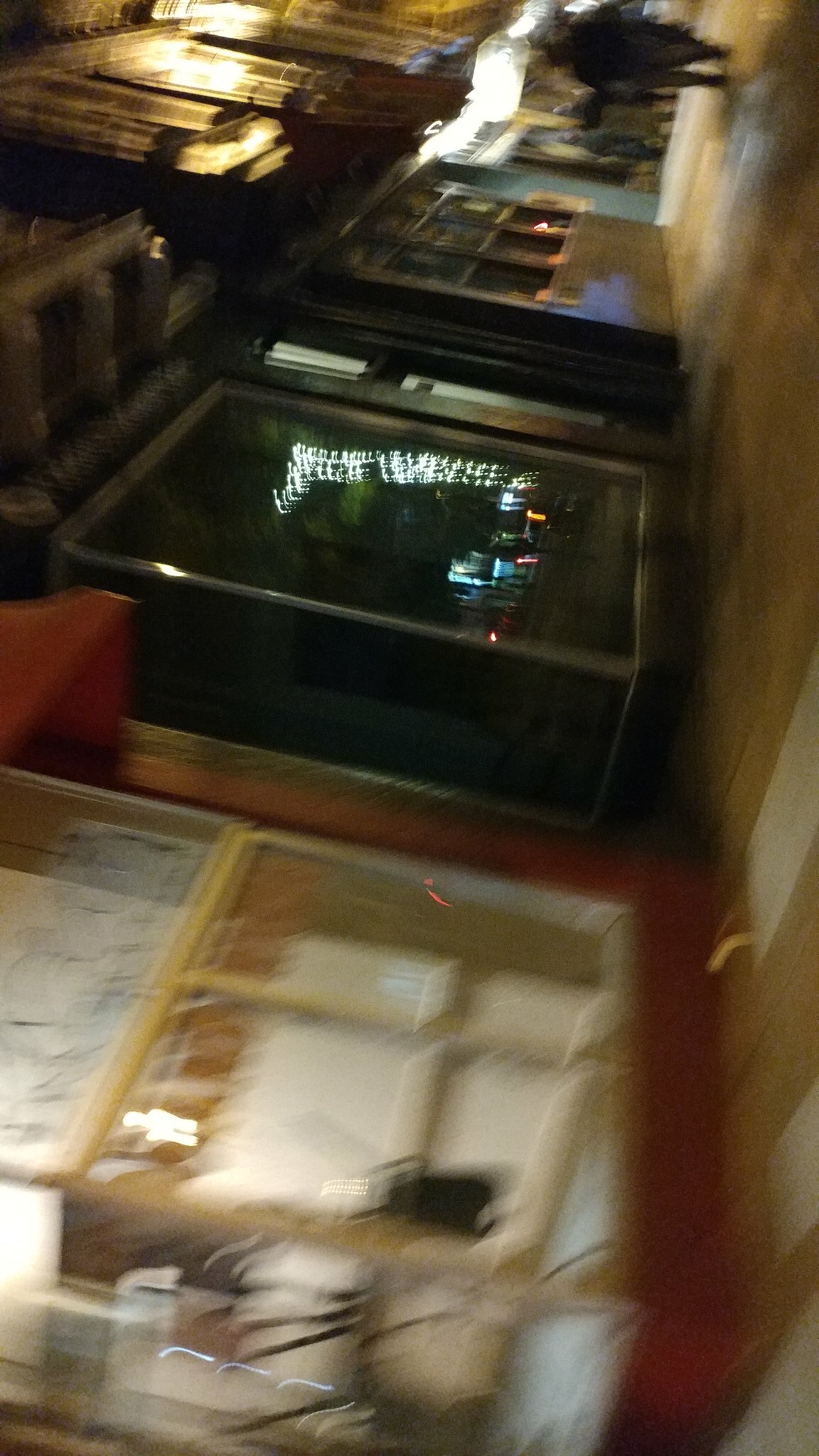This photograph, although very blurry and out of focus, depicts a nighttime city street scene taken from a disorienting 90-degree angle. The storefronts line the top of the image with their doors and windows facing upwards, while the sidewalk occupies the right side, creating an unusual perspective. The image suggests a commercial area, perhaps a shopping center, featuring several windows displaying reflections of festive lights, potentially Christmas lights, indicating it's nighttime. A distant group of people can be partially seen walking on the sidewalk. One window hints at an interior view, possibly of a closed cafe or restaurant, as chairs are stacked upside down on tables. The sidewalk appears to be tiled in brown and white patterns. Despite speculation in the descriptions about indoor showrooms or model displays, the overall consensus leans towards an exterior street view with a close-up on the storefronts and their reflections.